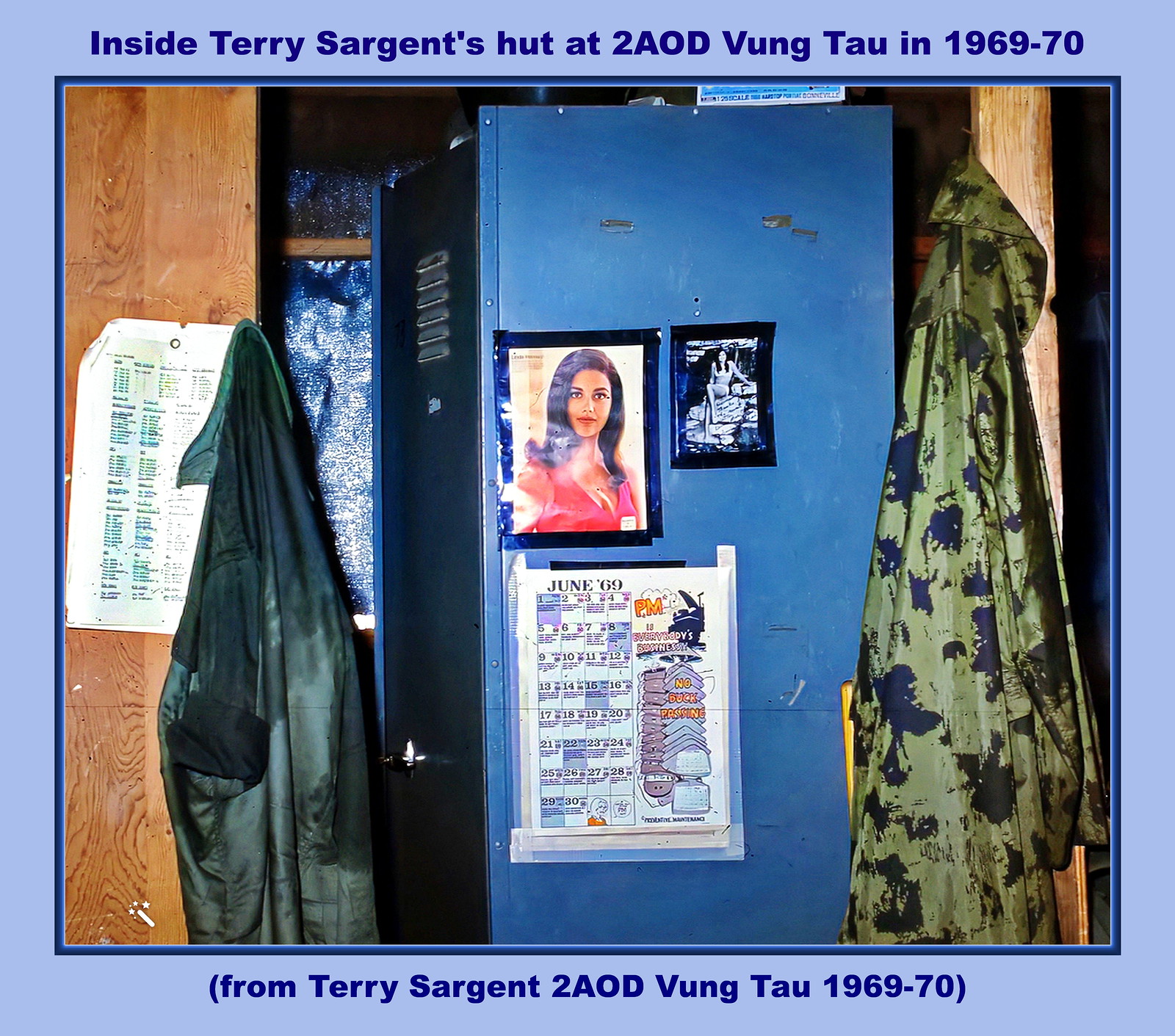The image captures the interior of Terry Sargent's hut at 2AOD Vung Tau in 1969-70. A blue metal locker, adorned with photos and posters, is prominently featured. Taped to the locker are pictures of two dark-haired women, one in a pink tank top and another seated on a chair, alongside a white schedule from June 2009 with blue text. The closely positioned wooden closet, with a white piece of paper thumbtacked on it, frames the locker. A black jacket hangs from a hook on the left door, while a green and black camouflage jacket dangles from the right. The photo is bordered by a light blue frame with a dark blue inset line. Both the top and bottom of the photo contain dark blue text identifying it as "Inside Terry Sargent's Hut at 2AOD Vung Tau in 1969-70" and attributed to Terry Sargent.